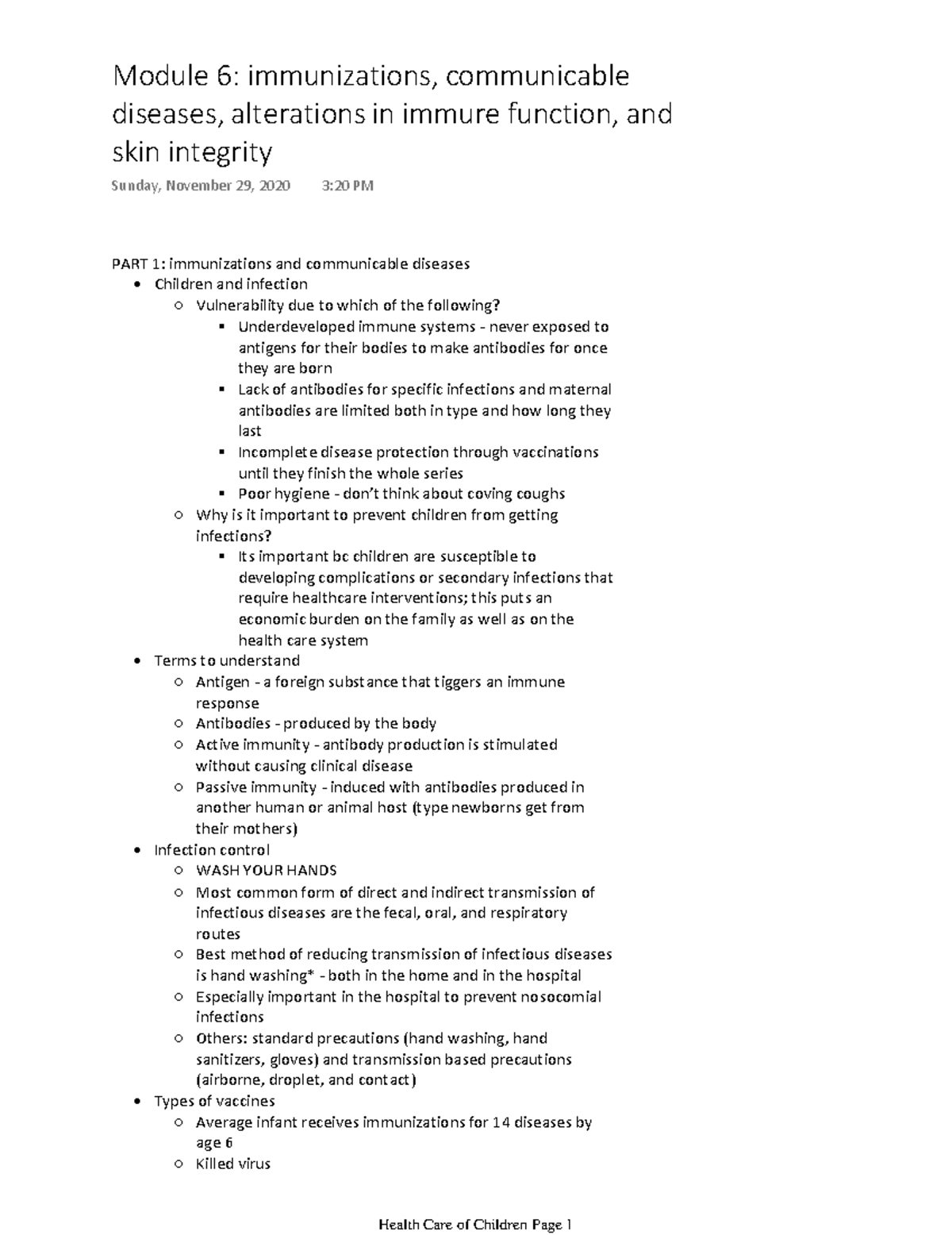**Module 6 Overview: Immunizations, Communicable Diseases, Alterations in Immune Function, and Skin Integrity**

**Date & Time:** Sunday, November 29, 2020, at 3:20 PM

**Part 1: Immunizations and Communicable Diseases**

**Key Topics Covered:**

1. **Children and Infection Vulnerability**
   - Underdeveloped immune systems at birth.
   - Lack of exposure to pathogens leading to minimal body antibodies post-birth.
   - Maternal antibodies' limitations in providing specific infection protection and uncertainty about their duration.
   - Incomplete disease protection until vaccination series are fully completed.
   - Importance of avoiding infections to prevent complications and secondary infections, thus reducing healthcare intervention needs and economic burden on families and the healthcare system.
   - Mechanisms of the immune response, including the production of antibodies.

2. **Types of Immunity**
   - **Active Immunity:** Stimulated antibody production without causing clinical disease.
   - **Passive Immunity:** Introduction of antibodies produced by other humans or animal hosts, crucial for newborns.

3. **Infection Control Practices**
   - Hand washing as the most effective method to prevent the transmission of infectious diseases through fecal, oral, and respiratory routes.
   - Emphasis on regular hand washing both at home and in hospital settings to reduce the risk of infections.

This detailed overview underscores the intricacies of managing children’s immunizations and understanding the variables that contribute to their vulnerability to infections. Proper hygiene practices, especially hand washing, remain a cornerstone for preventing the spread of diseases.